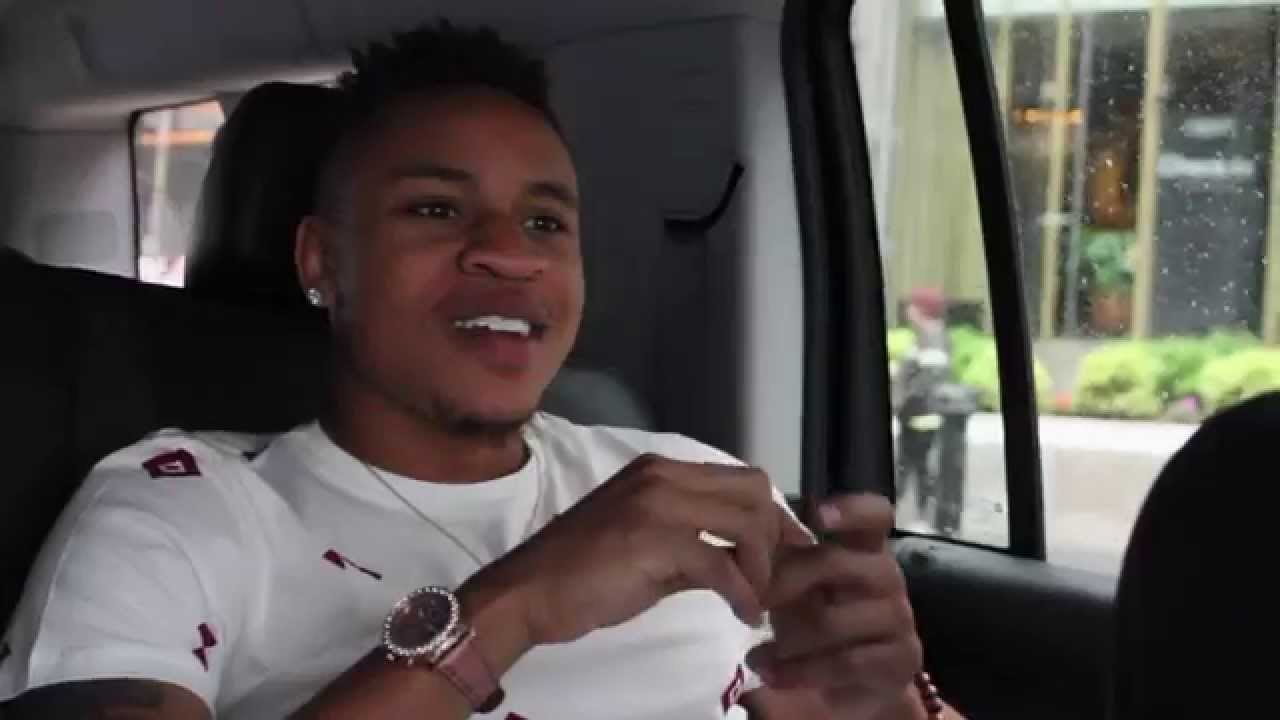This is a close-up photograph of a young African-American man sitting in what appears to be the back seat of a car, likely on the driver's side. He has short, curly black hair styled with the sides shaved and the top raised, creating a mohawk-like effect. He sports a small smile, revealing bright white teeth, and has a diamond earring in his right ear. He is wearing a white short-sleeved shirt adorned with several small red geometric designs, including a diamond shape on his shoulder and an hourglass on his arm, although one design near the collar is obscured by a fold. Around his right wrist, he wears an elegant analog watch with a pink or tan leather band and a face encrusted with jewels. His hands are visible and appear to be clasped together. The car window next to him shows droplets of water, indicating it might be rainy outside. Through this window, a slightly blurred view of the outdoors reveals a building with a yellow-framed window and some bushes on a cement platform. Additionally, there’s a man outside wearing a red hat and a black jacket with yellow accents. The overall setting, both inside the car and the glimpse of the exterior, suggests a city environment.